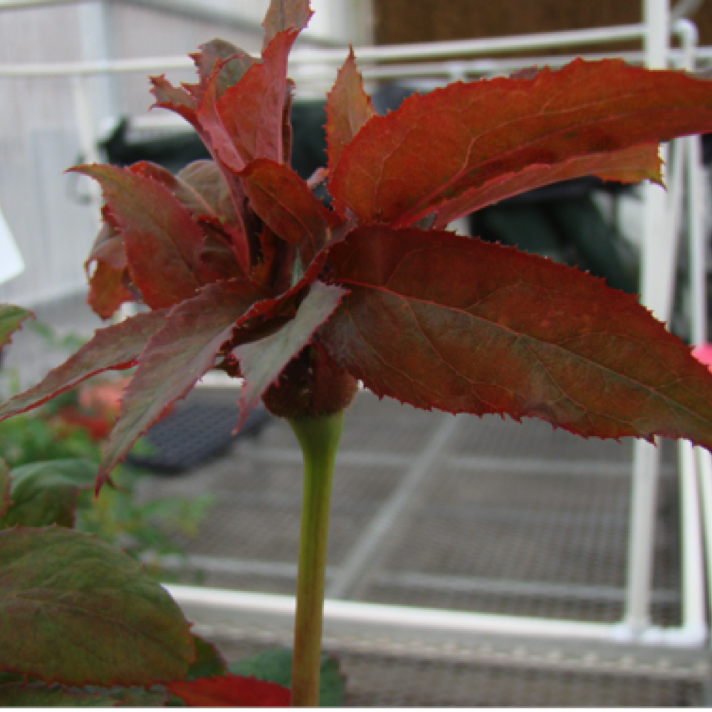The image features a close-up shot of a collier flowering plant, centered on a thick, green stem that extends from the bottom towards the middle of the frame. The top of the stem is crowned with a cluster of predominantly burgundy and autumn-colored leaves, showing a mix of red and green hues with jagged edges that appear torn. Some leaves exhibit small brown spots, suggesting they might be aging as the chlorophyll drains. Surrounding the main stalk are green leaves from other collier plants. The background consists of a blurred, gray floor and white poles, likely indicating a controlled environment such as a greenhouse. The overall ambiance conveys a vibrant autumn setting, enhanced by the contrast of colorful foliage against the muted backdrop.